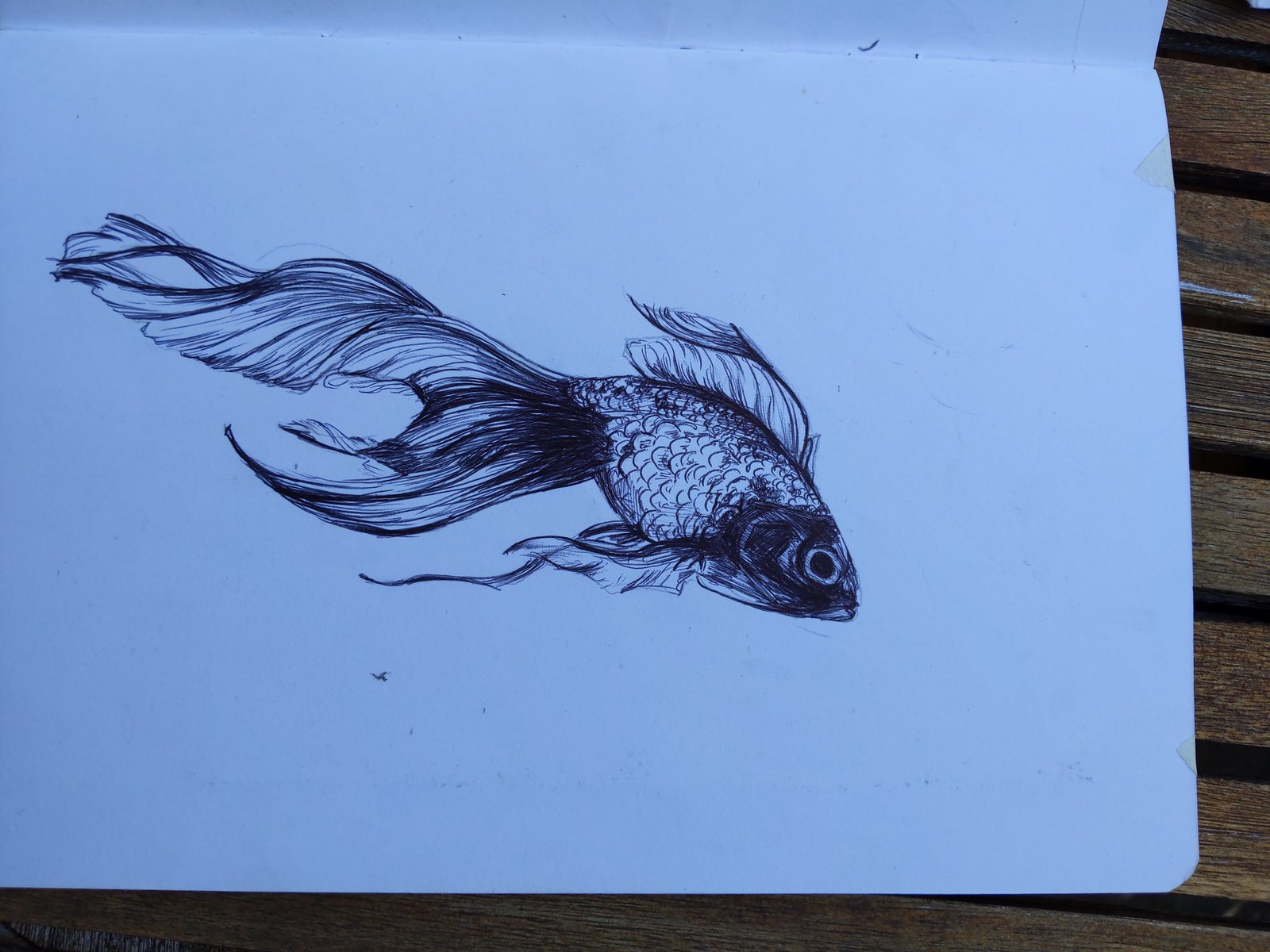This highly detailed pen and ink drawing portrays a koi fish captured in profile, elegantly rendered in shades of black and grey. The intricacies of the drawing reveal individual scales meticulously illustrated across the fish's body. The koi’s top fin, slightly coiled down, contrasts with its elongated and dangling lower fin. Its elaborate tail fin extends far beyond the length of its body, creating a sense of graceful motion as it slants downward on the page. The drawing is presented on a wooden slatted surface, lending a rustic backdrop to the artwork. A subtle, bluish light bathes the scene, imparting an indigo to navy wash over the image, adding a touch of mystique to the solitary fish.